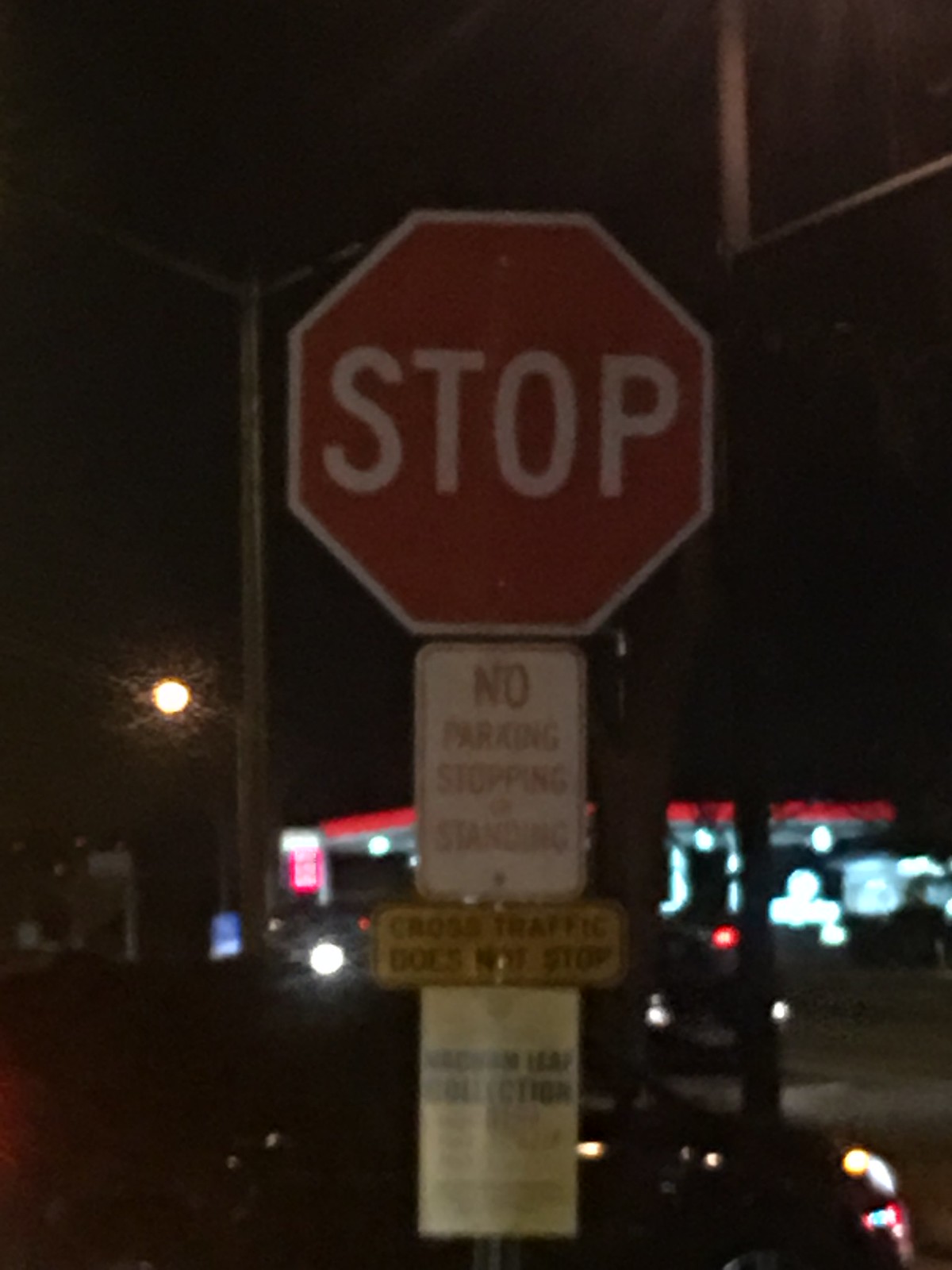The photograph captures a nighttime scene centered around a stop sign in the foreground. The red octagonal stop sign is prominent, with several other signs affixed to its pole. Directly beneath the stop sign, a red and white rectangular sign clearly states "No Parking, Stopping, or Standing." Below this, another white rectangular sign reads "Cross Traffic Does Not Stop." A third, lighter-colored sign is further down the pole, but its text is illegible due to blurriness.

In the background, a brightly lit structure, likely a gas station, is visible. The gas station features a red and white sign and a red roof or canopy, although the details are somewhat obscured by the distance and the blurred quality of the image. The overall scene is enveloped in darkness, with the illumination from the gas station providing the primary light source.